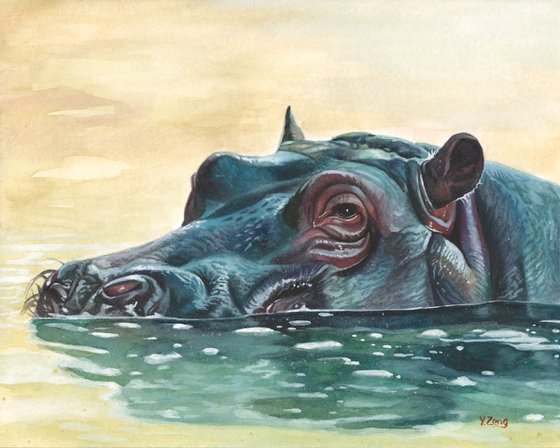The image is a detailed, watercolor painting of a hippopotamus titled and signed by the artist "Y. Zong." The hippo, predominantly painted in shades of blue and aqua with accentuating reds, appears half-submerged in a lake. The central focus is on the head and neck of the hippo, which is facing leftward. Notable features include its large, dark gray nostrils just above the water surface, with hair-like details around one of them, and its single visible, deeply dark eye framed by red and brown wrinkles. The cute, round ears, also tinged with red, contrast against its overall skin texture that hints at the effects of water. The water surrounding the hippo reflects various blended hues of blue, teal, and green, transitioning to a yellowish tan towards the background, possibly indicating sunlight reflection. The hippo's shadow beneath the water is depicted in dark gray tones, lacking specific details but adding to the composition's depth. The scene captures the serene and natural essence of the hippopotamus, highlighting its calm presence within its aquatic environment.